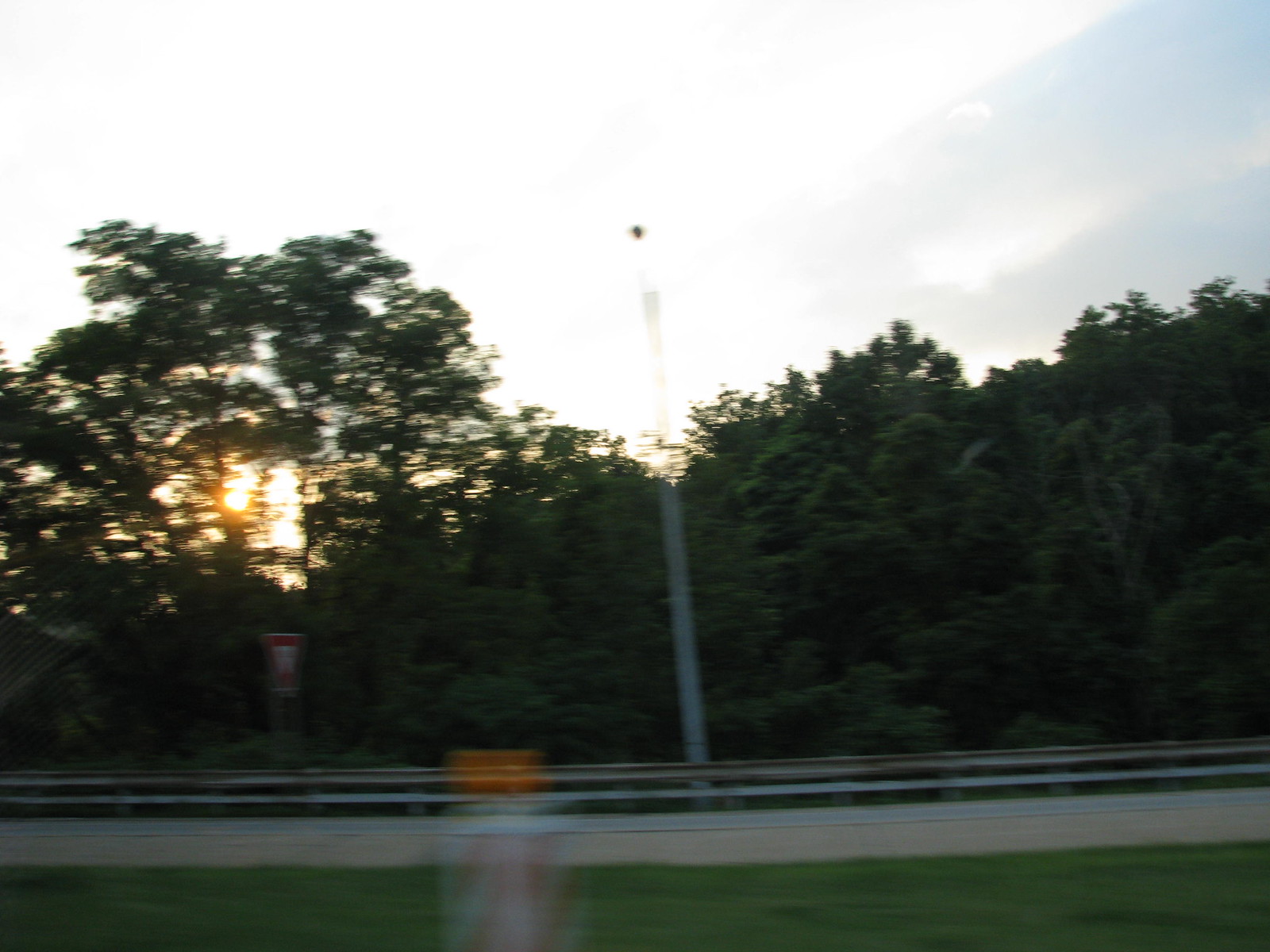The photograph, capturing a scene from inside a car, features a subtle window reflection near the lower center, possibly revealing a can with an orange top. The primary focus of the image is a roadside view. Dominating the lower portion is a guardrail, leading up to a pole situated centrally in the frame. In front of the guardrail, a patch of grass provides a vibrant foreground element. The background is densely populated with trees, with an especially tall, somewhat see-through tree on the left. Sunlight streams through the trees, adding a natural glow to the scene.